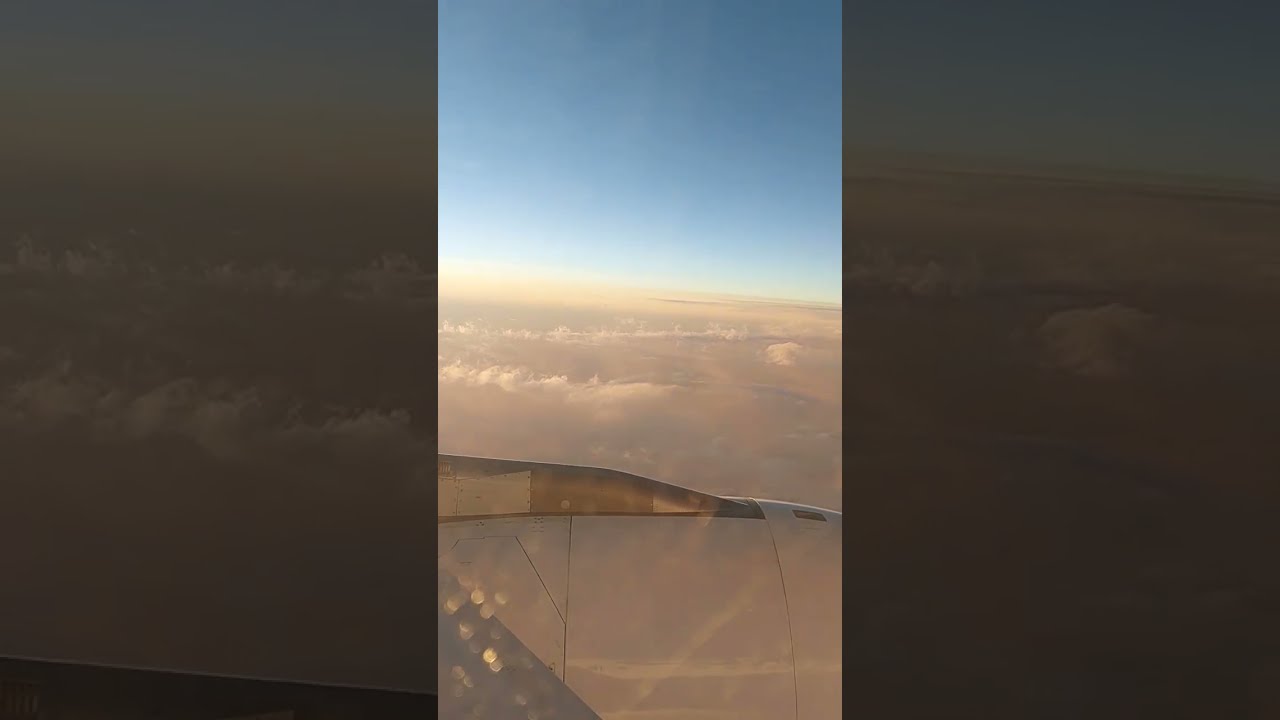This image, captured from a passenger jet approaching London, primarily showcases the view from a high elevation. The viewer's perspective is from the airplane window, framed vertically as a cell phone photograph. Dominating the foreground is the circular cylindrical engine beneath the fairing, distinctly visible with its red and silver hues. Above, the pure blue sky serves as a serene backdrop. Below, thin, wispy tan-colored clouds drift over a vast, barren landscape that resembles a desert, stretching far into the horizon. The scene suggests a mid-afternoon timeframe, bathed in subtle sunlight. While the background is a blurred and zoomed-in version of the main picture, the overall composition maintains a sense of anticipation as the plane descends towards London.